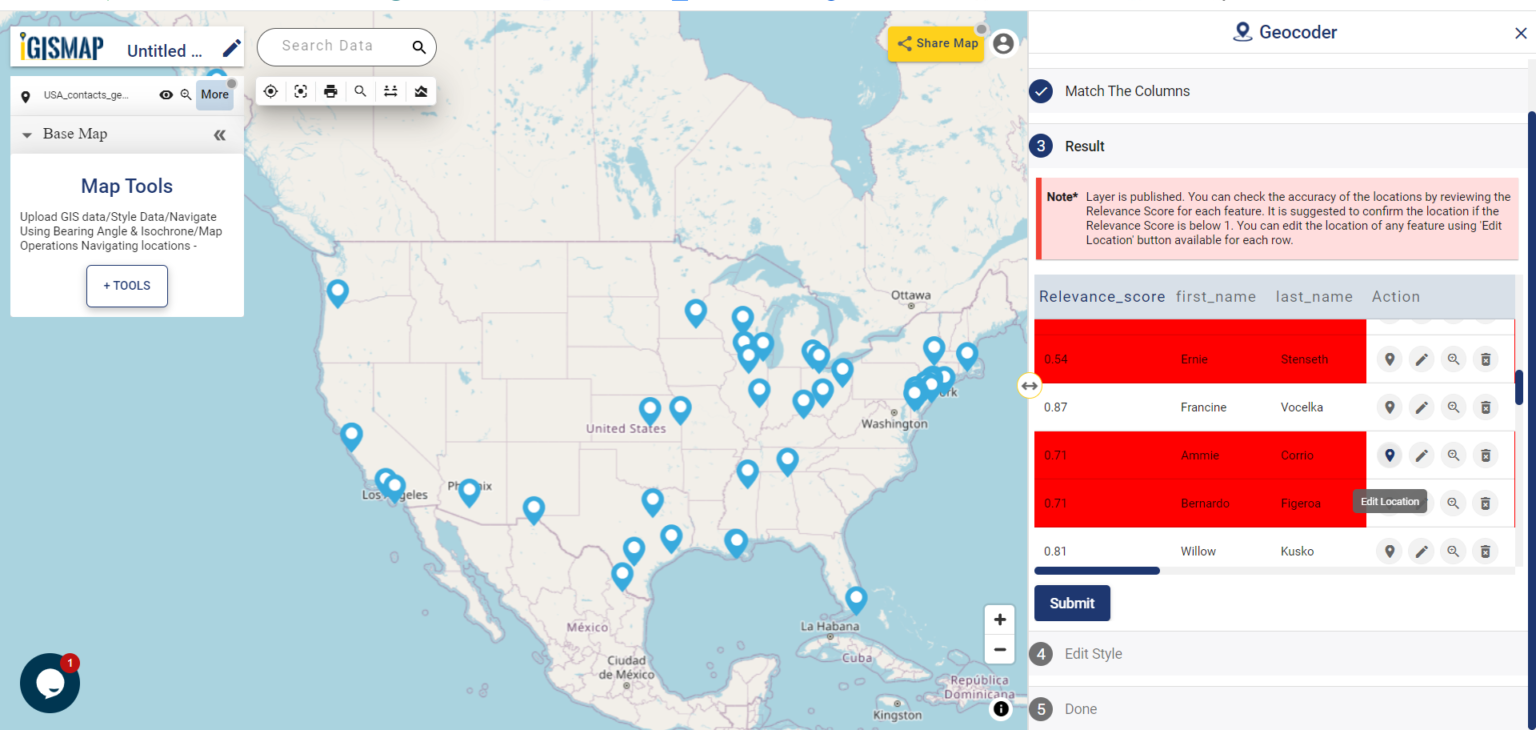**Detailed Caption for GIS Map Application Screenshot:**

The screenshot showcases an interface from a Geographic Information System (GIS) map application. On the left side of the screen, the header displays "GISMAP." Below it is the title "untitled..." accompanied by a pencil icon, suggesting that the title is editable. Beneath that, the text reads "USA_contacts_GE..." with an eye icon and a search icon adjacent to it, and the word "more" highlighted, implying additional options or layers are available. Next, a section labeled "base map" features a caret indicating it can be expanded.

Further down, there's a white toolbox labeled "Map Tools," with functionalities like uploading GIS data, using bearing angles, and isochrone mapping. The second line describes navigation and map operations for locations. Following this, a box with a plus symbol labeled "Tools" is visible.

The central part of the screenshot displays a map with a blue oceanic background, depicting the countries of the United States, Canada, and Mexico. Multiple blue pointers with white centers are distributed across various locations, indicating key points or cities. Notably, three pointers are in California, one in Oregon, one in Kansas (above Oklahoma), four or five in Texas, and several others distributed across states like Louisiana, Alabama, Mississippi, Kentucky, Ohio, Illinois, Michigan, Idaho, and along the East Coast from Washington up past New York City.

On the right side of the screen, the header "Geocoder" is prominent, with rows labeled "match the columns" and "Result." Below this, a light red note states: "Layer is published. You can check the accuracy of the location by reviewing the relevance score for each feature. It is suggested to confirm the location if the relevance score is below one. You can edit the location of any feature using the edit location button available for each row."

Below this note, a table is present with headings: "relevance_score," "first_name," "last_name," and "action." The first entry in the table shows a relevance score of 0.54 for "Ernie Sternseth," highlighted in red, with action icons including a location marker, pencil, search icon, and an unidentified icon. Subsequent entries include "Francine Vocelka" with a score of 0.87, "Amy Corio" at 0.71, "Bernardo Figueroa" also at 0.71, and "Willow Cusco" at 0.81, all accompanied by the same set of action icons.

The interface suggests scrollability for more entries and provides navigation options. A blue "submit" button is seen below the scrollable area. Sections labeled "4. Edit style" and "5. Done" are grayed out, indicating they are currently inactive.